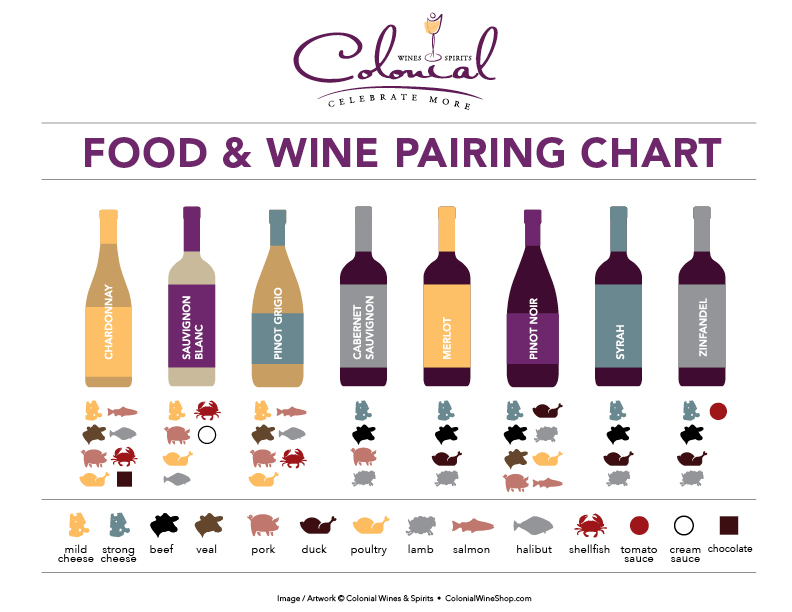This image is an advertisement for Colonial Wines and Spirits, featuring a detailed food and wine pairing chart from colonialwineshop.com. At the top of the image, the title "Wine and Spirits" is prominently displayed in black lettering, while just below, the phrase "Celebrate More" is written in elegant purple cursive. The main section of the chart showcases eight different bottles of wine, each in a distinct color ranging from yellowish peach to deep purple, blue, dark gray, and almost black. Each bottle is labeled with its respective type of wine: Chardonnay, Sauvignon Blanc, Pinot Grigio, Cabernet Sauvignon, Merlot, Pinot Noir, Syrah, and Zinfandel.

Directly beneath each wine bottle, a series of symbols represent various foods that pair well with the respective wines. The symbols illustrate an array of foods including crab, halibut, salmon, lamb, poultry, duck, pork, veal, beef, cheese, shellfish, tomato sauce, cream sauce, and chocolate. For instance, Chardonnay pairs excellently with mild cheese, veal, pork, poultry, salmon, halibut, shellfish, and chocolate. Similarly, Sauvignon Blanc complements cheese, shellfish, cream sauce, pork, poultry, and halibut, whereas Cabernet Sauvignon aligns best with strong cheese, beef, pork, and lamb. 

The image provides a comprehensive guide for pairing each type of wine with suitable dishes, accentuated with pictograms for easy reference and a visually appealing display, aiding wine enthusiasts in making informed pairing decisions.